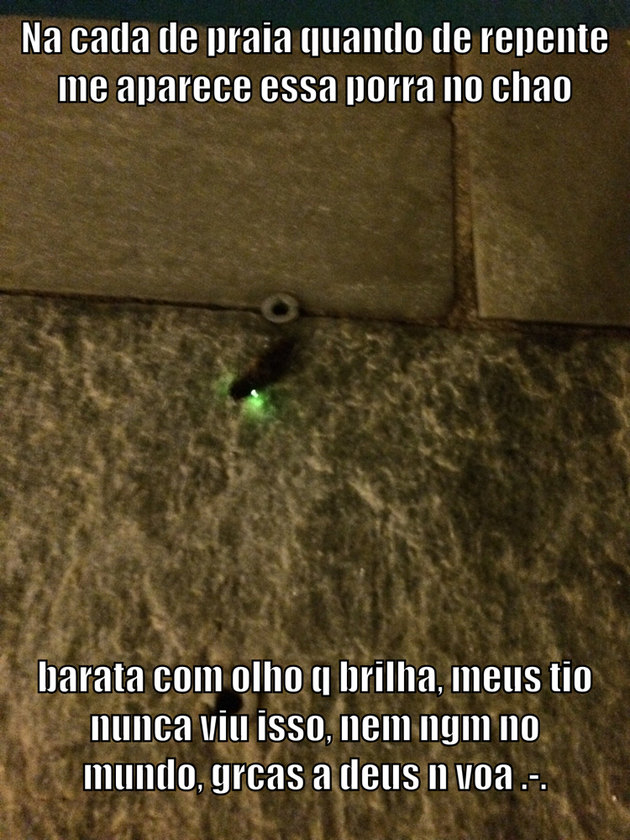The image is a confusing close-up of a medium brown, yellowish-brown, and gray construction material, possibly ceramic tile or brick. The surface is partially illuminated, revealing a small, black, hooked pipe or object that emits a neon green glow from its end, which could resemble a door stopper or a screw set within a concentric circle border. The background texture suggests a rougher, more textured concrete or structural element underneath the smoother upper surfaces. Superimposed on the image is text in white font, in what appears to be Spanish, with two lines at the top saying "Nakata de prior cuando de repente me apreque esa porra no cao" and three lines at the bottom, albeit unclear, suggesting "Barata como alto que brilla mustio nunca vi su hosi".